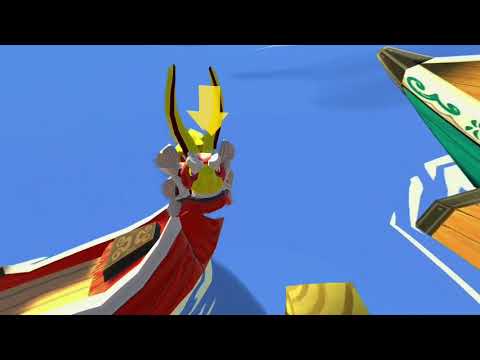The image appears to be a screenshot from a video game, showcasing the bows of two computer-rendered boats floating on solid blue water. On the left, there is a boat with a red hull and white trim. The bow features a striking crest resembling an oriental mask or dragon head, adorned with long vertical yellow and black horns, white eyebrows, and a distinctive yellow nose. A yellow arrow points down toward this dragon head. To the right is the bow of another boat, which is green with white trim and green patterns. The interior seems to be light tan wood. Additionally, there is a golden shape in the bottom right, though it is unclear what it is connected to. The image is framed by black bars running along the top and bottom, and the left side of the second boat has a light teal green hull with a black tip at the front. Both boats are depicted on a solid blue background, which suggests a simplified representation of water.